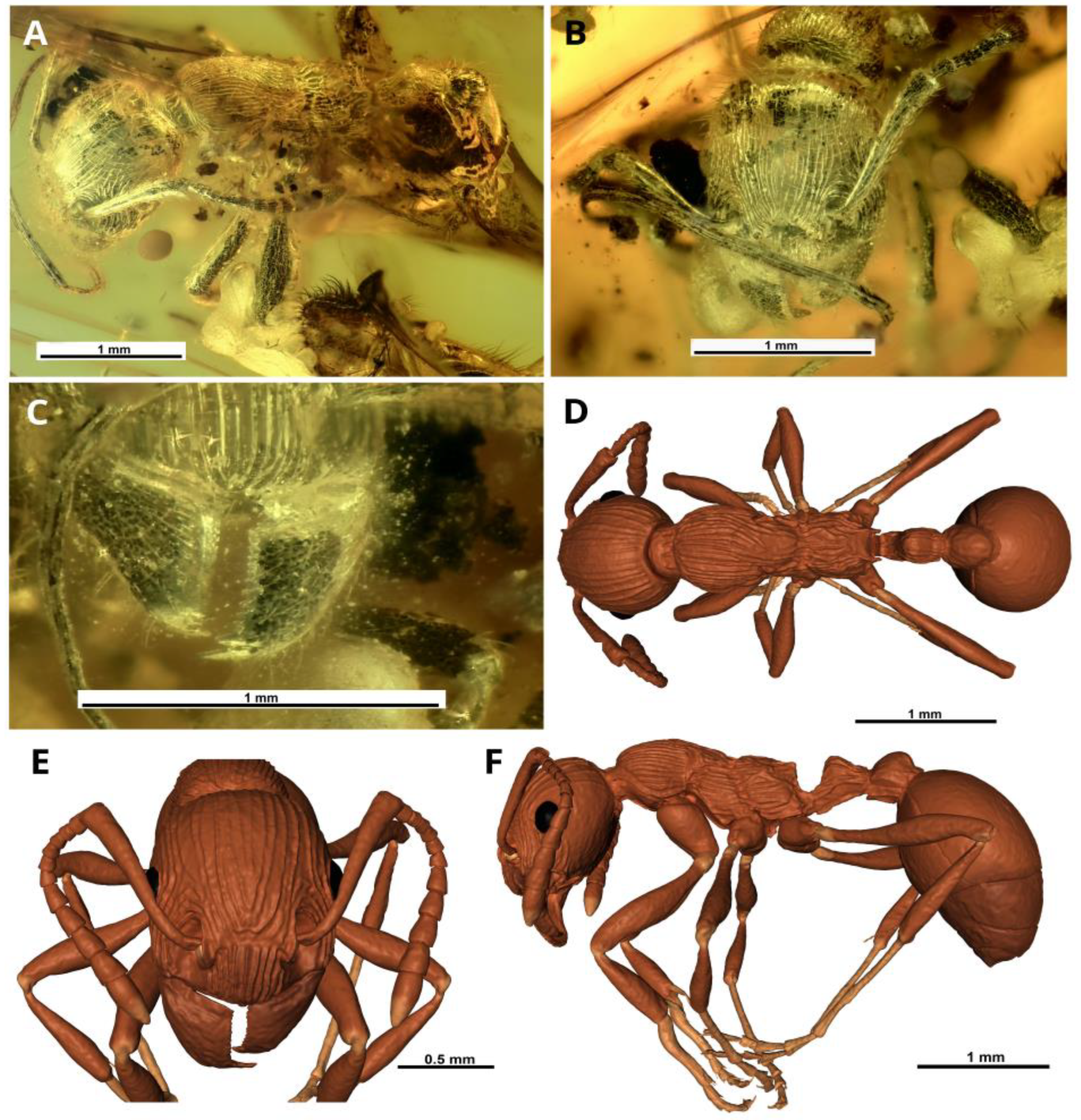The image is a comprehensive study of an insect, likely an ant, displayed as a combination of photographs and illustrative charts. The set is arranged into six distinct sections labeled from A through F. The top three images (A, B, and C) are full-color photographs capturing different perspectives of the ant. Picture A provides an overview of the ant's body, Picture B offers a slightly closer view focusing on the head, and Picture C is a close-up of the ant's head. The lower three images (D, E, and F) are detailed, black-and-white illustrations. Picture D shows an overhead shot of the ant's back, Picture E presents a frontal view highlighting the head and antennas, and Picture F depicts a side view detailing the legs, head, thorax, and abdomen. Each image includes a scale notation, mostly indicating one millimeter, while one shows a scale of 0.5 millimeters, giving an indication of the magnification and actual size. The blend of real photographs and diagrams offers a thorough visual examination of the ant from multiple dimensions and developmental stages.